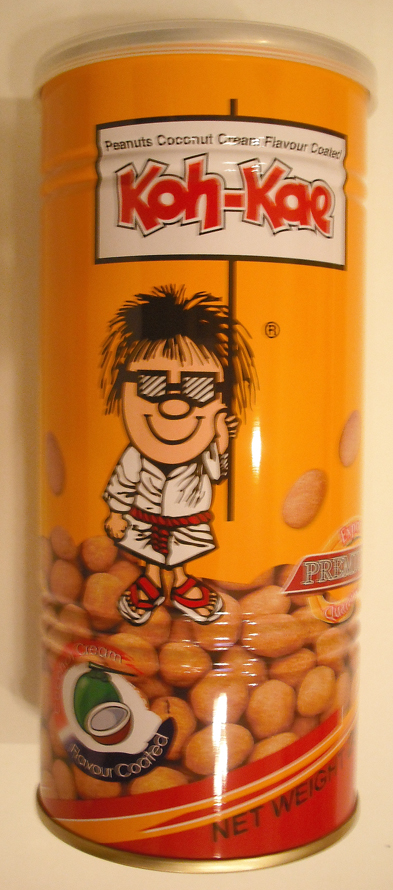The image depicts a brightly colored orange tin container of flavored snacks. The container prominently features the brand "KOH-KAE" at the top, indicating that it holds coconut cream-flavored coated peanuts. A whimsical cartoon character, a boy dressed in a white martial arts uniform and sporting black sunglasses with white lenses and black stripes, is shown holding a sign that describes the product. The container is adorned with appetizing images of the peanuts, which are highlighted and described as premium quality and creamily coconut cooked. The playful design and bold presentation make the product stand out.